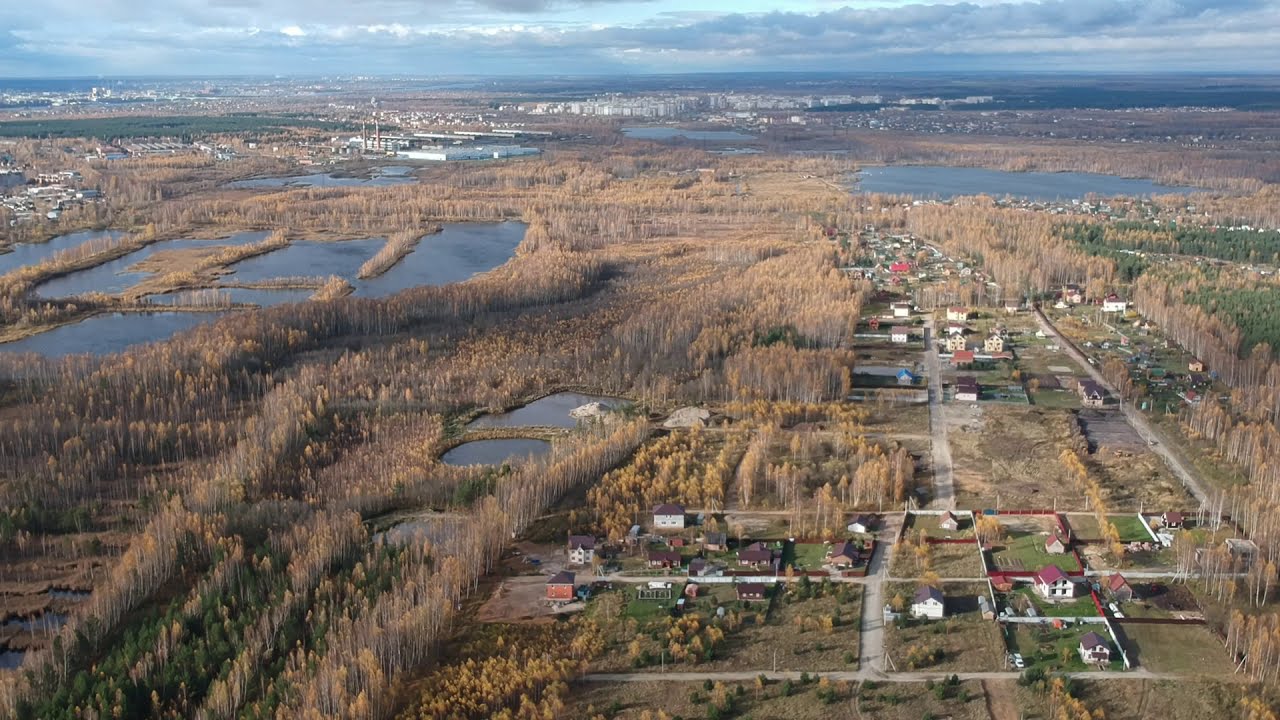This aerial image captures a small village under a clear, blue sky with scattered white clouds. The landscape is dominated by high grass and a series of water bodies, including ponds and bogs, which give a hint of Everglades or swampy characteristics. The trees throughout the image are predominantly brown and yellow, suggesting a fall or late autumn scene. Further off, the village is visible with its array of white buildings. 

In the lower right corner, a residential neighborhood is showcased, consisting of houses with red and gray roofs and white or reddish brick sidings. The streets surrounding these houses contain various cars, forming a neat grid of parcels. The overall setting is sunlit, enhancing the earthy, winter-like tones of the environment. Bright patches of green and yellow trees intersperse the brown grass, adding a touch of color to the serene, nature-infused scenery.